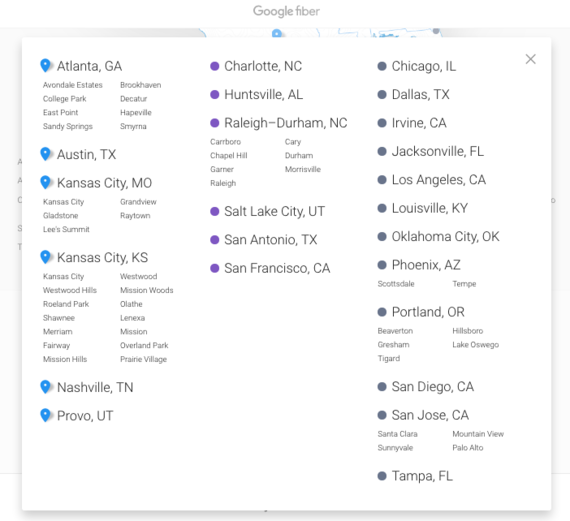The top of the image displays the title "Google Fiber." On the left side, there's a list of locations starting with "Atlanta, Georgia," and including places such as Blue Pin, Dallas, Chase, Brookhaven, College Park, Decatur, Peace Point, Hapeville, Sandy Springs, and Marina. It also mentions "Purpose of Charlotte, NC," and extends to Highline, Dachshund, MIT, Canberra, Chapel Hill, Gardner, Raleigh, Cary, Durham, Monsal, Chicago, Illinois; Charlotte, Texas; Irvine, California; Jacksonville, Florida; Los Angeles, California; Louisville, Kentucky; Oklahoma City, Kansas City, Kansas; Kansas City, Westwood Hills; Westwood, Bishopwood, Sola; Lenox, Shawnee, Marina; Mission, Fairway, Overland Park; Michelle's Village; Nashville, Kansas City; Poverty. 

On the far right side of the image, the list includes locations in Portland, Oregon; Beaverton, Ellsworo, Gretchen Lake, Osogo, Tigard; San Diego, California; San Jose, California; Santa Clara, Mountain View, Sunnyvale, Palo Alto; and Tampa, Florida.

Perhaps these are the locations where Google Fiber is available.